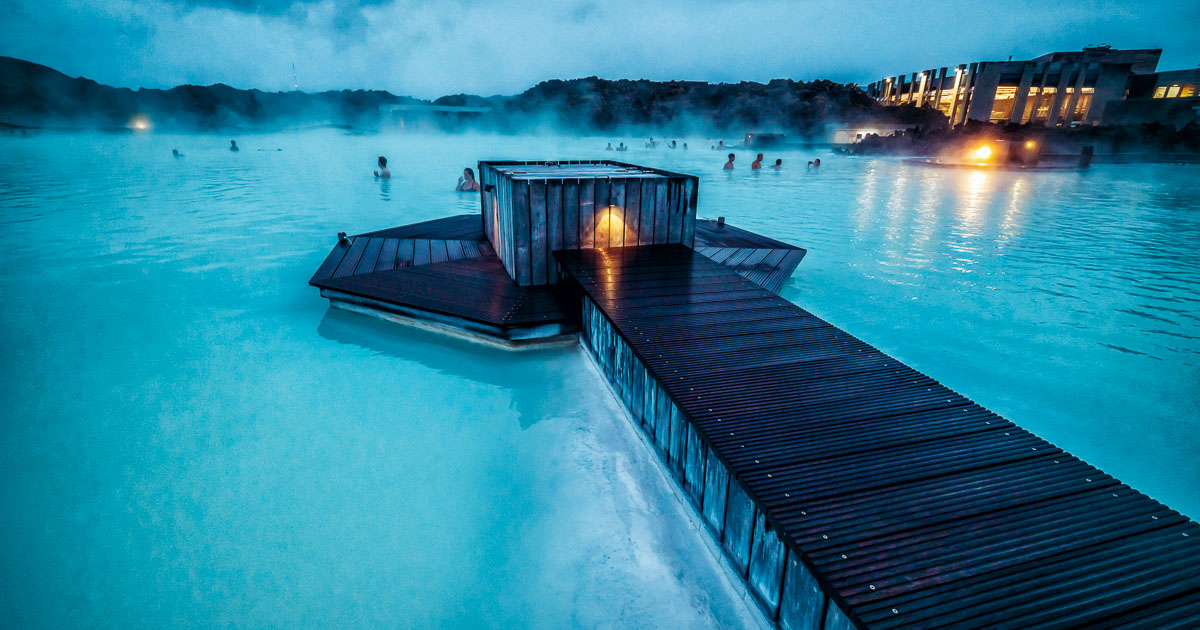This image captures a tranquil nighttime scene of what appears to be a large, serene hot spring or lagoon, possibly the Blue Lagoon. The body of water dominates the image with its striking, clear aqua blue and light steam rising from its surface, suggesting it is heated. 

In the foreground, a wooden pier extends about 10 yards out into the water and culminates in an octagonal platform. Atop this platform stands a small, square box-like structure emitting an orange light, reminiscent of a lantern or illuminated window. The structure, which possibly resembles a storage container made of picket-fence-like material, adds an intriguing and mysterious element to the scene. 

Scattered throughout the water are several people, swimming or wading, which enhances the impression that this location might be a resort or a recreational spot. The presence of mist or fog hanging in the air further adds to the mysterious and esoteric atmosphere.

In the background, you can see a large, well-lit building that could be an industrial structure, hotel, or resort, perched on or near hills. The land behind is silhouetted against a darkening sky that mirrors the color of the water, while dark mountains or hills frame the scene, with wispy clouds or possibly more steam adding to the mystical ambiance.

Overall, the image evokes a sense of peace and calm, capturing the serene beauty of this possibly resort-like location.